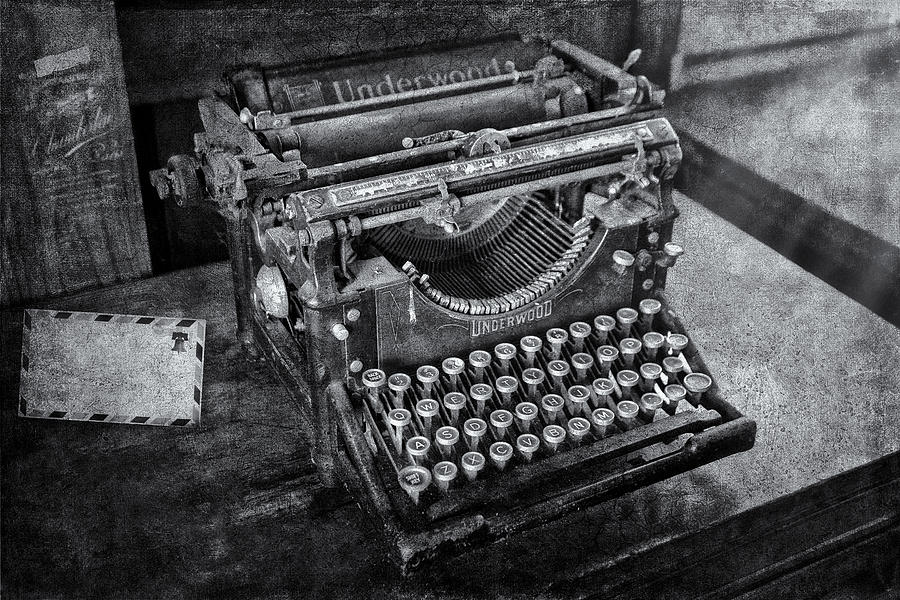This black-and-white, grainy photograph captures a vintage Underwood typewriter, angled counterclockwise about 45 degrees on a wooden desk. The typewriter, with its distinctive round keys and labeled letter and number buttons, prominently displays the "Underwood" branding above and below the keystrikes. To the left of the typewriter lies a white envelope bordered in a black-and-white checker pattern, featuring a stamp of the Liberty Bell. In the background, behind the typewriter, there appears to be an open book or advertisement, with some obscured white lettering visible. The image's graininess adds to the nostalgic ambiance, evoking a bygone era of analog correspondence and manual typing.